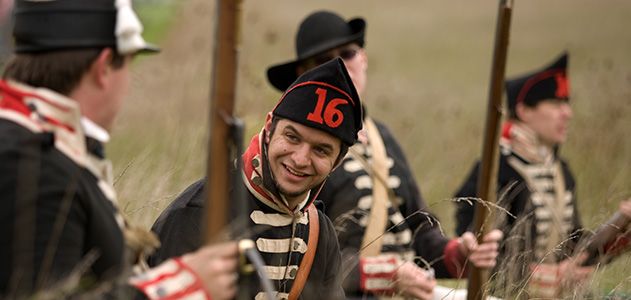This photograph captures four men standing in a golden wheat field, dressed in black military uniforms adorned with cream-colored horizontal stripes and gold fabric trims running parallel from the neck to the waist. Their attire is reminiscent of American Civil War-era uniforms, complete with black hats featuring the number "16" in red. Each man carries a rifle, with the wooden stocks clearly visible. The focus is on one man whose face is turned toward the camera, smiling at the man on his right. This central figure's expressive face conveys a sense of camaraderie. To his left, another man looks towards the central figure, though his face is not visible. Behind the central man, another soldier stands slightly blurred, adding depth to the scene. On the right, another man gazes out of frame. The background is dominated by the light golden hues of the wheat, with a small patch of green visible on the left, while the distant landscape remains blurry and indistinct, highlighting the timeless and nostalgic feel of the scene.